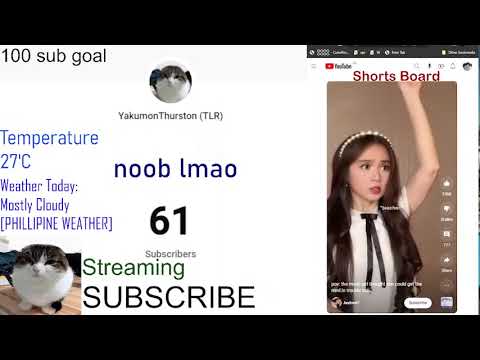The image features a central white background split into two distinct sections, framed by narrow black horizontal strips at the top and bottom. On the left side, there is diverse text and imagery. At the top left, in Arial sans-serif font, it reads "100 Step Gold," followed by a circular photo of a cat with a dark gray head, white chin, and cheeks. Below this photo, the username "Yakuman Thurston (TLR)" appears, accompanied by various pieces of colorful text: "Temperature 27 degrees Celsius," "Weather today: mostly cloudy, Philippine weather" (in purple letters), "noob lmao" (in blue), and "61 subscribers." Further text includes "streaming" in green and "subscribe" in black. 

On the right side of the image is a screenshot of a YouTube Shorts page, featuring a teenage girl, possibly Japanese or Korean, with long brown hair held back by a hairband. She is wearing a white top with a long black tie extending down the front and has her left arm raised, looking somewhat confused. Above her image, it reads "shorts board," with a small YouTube logo positioned above this text.